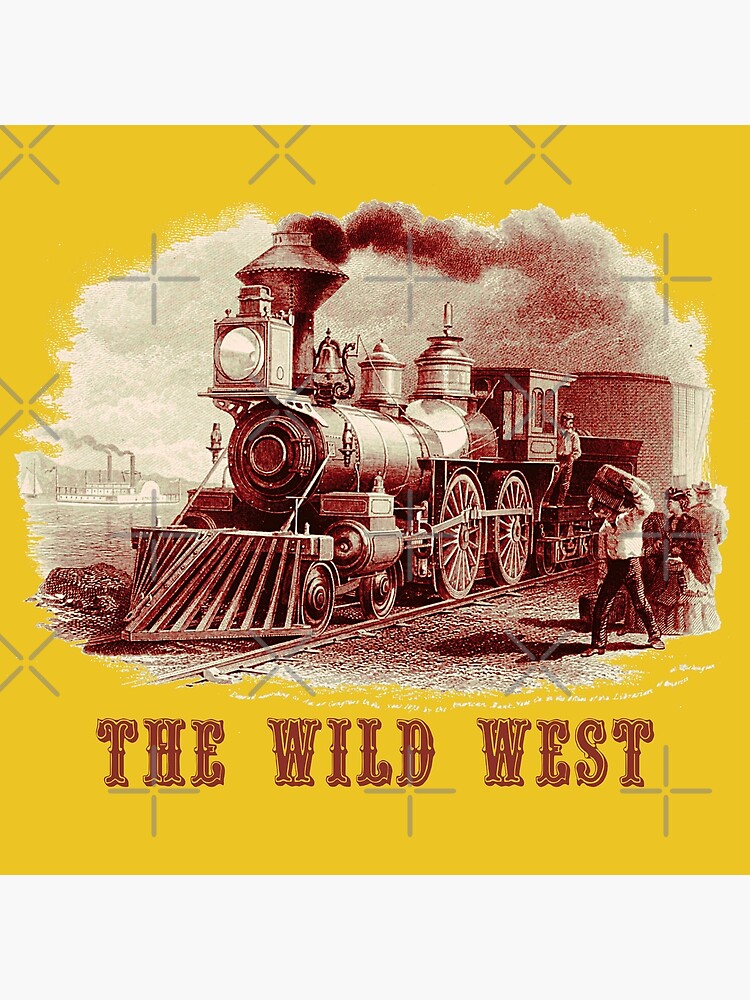This detailed hand-drawn image, resembling a vintage poster, showcases an old steam locomotive, rendered in a sepia tone mixed with reddish and dark ink. Set against a deep yellow background with gray crosses and hatches, the illustration prominently features the front engine car moving along the tracks. Smoke billows energetically from the smokestack while a large light and a cow catcher dominate the front of the train. The conductor is seen leaning out of the left side of the engine, and on the right, several people with luggage and cargo are depicted, adding a lively, yet desolate Old West town atmosphere. Behind the train, a steamboat can be faintly seen near a river, adding to the historical context of the scene. The image is completed with "The Wild West" written in old-timey, red lettering at the bottom.